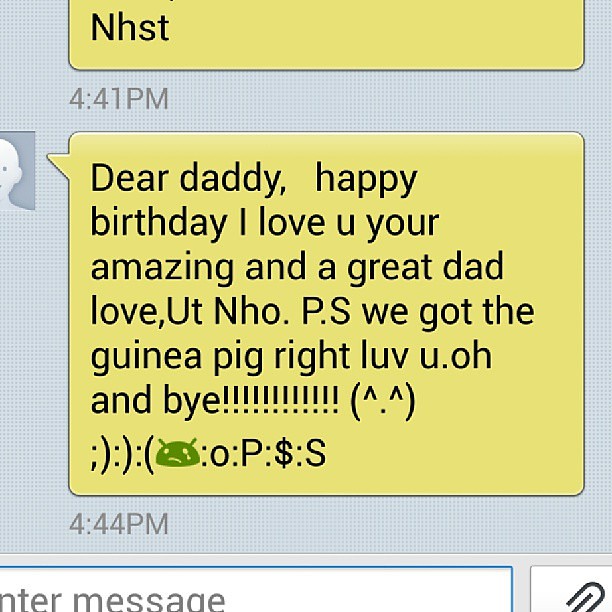The image is a screenshot of a text message conversation. The top part of the screen is cut off, showing only "NHST" partially visible. Below that, the timestamp "4:41 p.m." appears in gray font. The following yellow text bubble reads: "Dear Daddy, Happy Birthday, I love you, you're amazing, and a great dad, love, U-T-N-H-O-P-S. We got the guinea pig right. Love, U-O-N-I." This message is filled with various smiley faces and emojis, including an alien emoji, an 'O', a 'P', a dollar sign, and an 'S'. The next timestamp shows "4:44 p.m." Below the text input field, which is partly cut off, displaying "nter message," there are icons and symbols including a paper clip and a gray human face symbol.